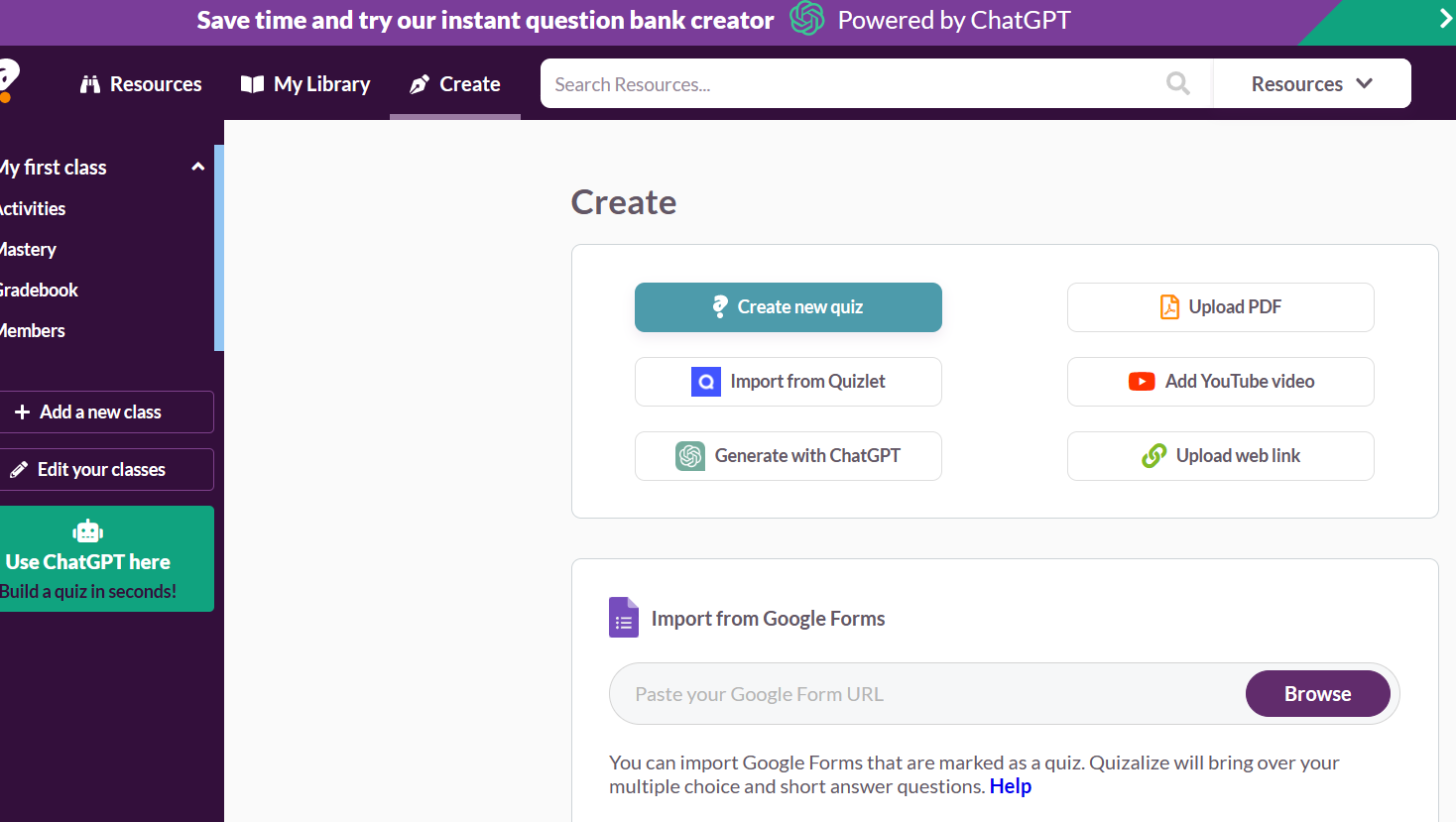This screenshot captures the interface of an online quiz-building platform. Dominating the top of the screen is a purple banner that reads, in bold white text, "Save time and try our instant question bank creator powered by ChatGPT." Just below this banner, spanning from left to right, are three navigation tabs: "Resources" accompanied by a binoculars icon, "My Library" marked with a book icon, and "Create" illustrated with a paintbrush icon. The "Create" tab is currently active, indicated by its highlighted state.

Adjacent to the "Create" tab, on the upper right, there is a search bar designed for finding specific resources. On the left-hand side of the page, a vertical sidebar menu offers a series of options: "My First Class," "Activities," "Mastery," "Gradebook," and "Members." Below these, there are additional options labeled "Add a New Class" and "Edit Your Classes." A prominent green box beneath this sidebar encourages the user to "Use ChatGPT here, build a quiz in seconds."

The central area of the "Create" page features six interactive buttons, each providing different functionalities. The buttons are labeled: "Create a New Quiz," "Import from Quizlet," "Generate with ChatGPT," "Upload PDF," "Add YouTube Videos," and "Upload Web Link." There is also an option for importing from Google Forms, accessible through a URL bar displayed further down the page. This detailed layout aims to streamline the quiz creation process, offering multiple pathways for educators to build and customize their quizzes efficiently.